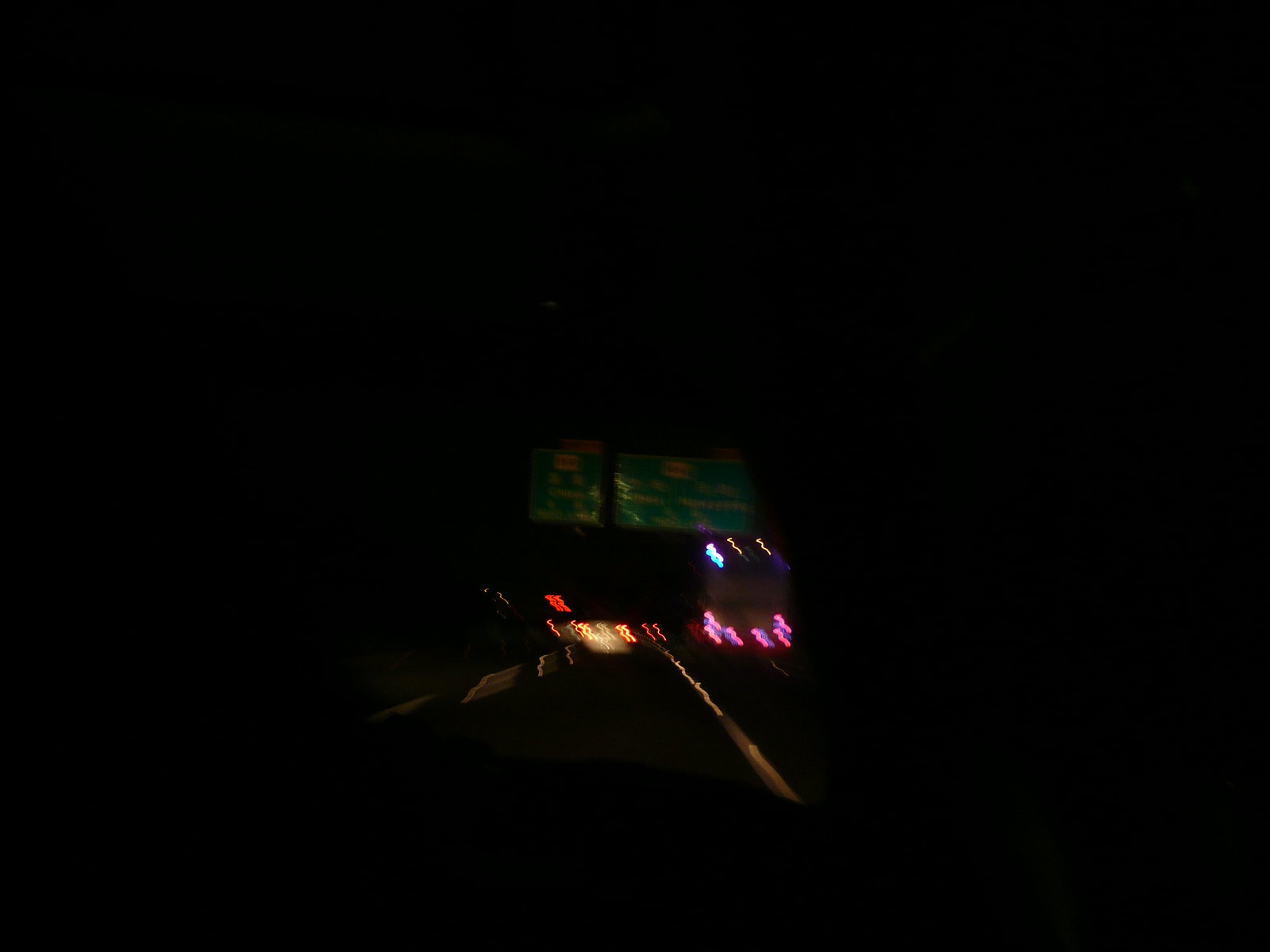This photograph captures a nighttime scene likely taken from inside a moving vehicle, as evidenced by its significant blurriness. The image appears to be shot with either a cell phone or a dashcam. The dark sky and shadowy elements within the frame confirm it was taken after sunset. Ahead of the car, another vehicle, possibly silver, is visible with its taillights glowing bright red. Additionally, on the right side of the image, there's another larger vehicle, which could be a bus or an RV, in a lighter color such as light gray or white. Above these vehicles, a pair of green highway signs with white writing can be seen, adding structural elements to the dark, motion-filled scene.